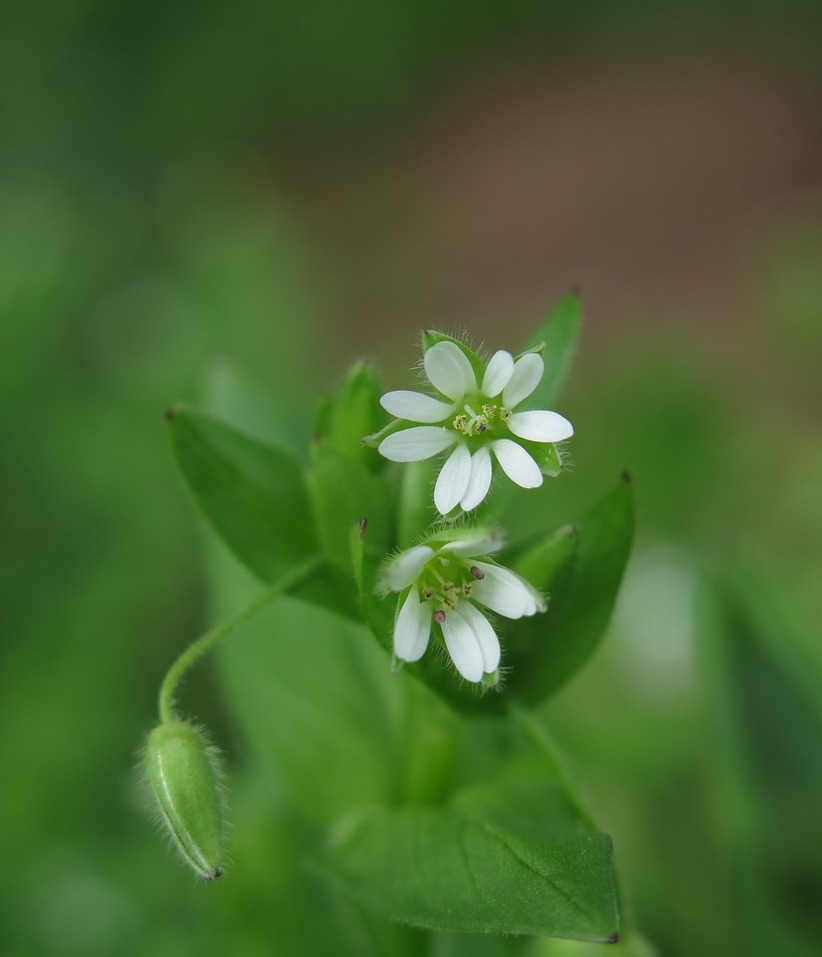This captivating close-up photograph showcases a delicate plant adorned with small white flowers. Each flower features ten oval-shaped petals arranged in pairs, encircling a fuzzy green center, providing a texture-rich appearance. The camera exquisitely captures the fine details, including the tiny fuzz that envelops the petals and leaves. Two flowers dominate the scene—one facing the viewer directly, while the other angles downward. Positioned to the left is a yet-to-bloom bud, pointing downward, surrounded by lush green leaves. The background is intentionally blurred, enhancing focus on the floral subjects and hinting at more greenery beyond. The overall composition highlights the intricate beauty and simplicity of nature in a soft, serene setting.